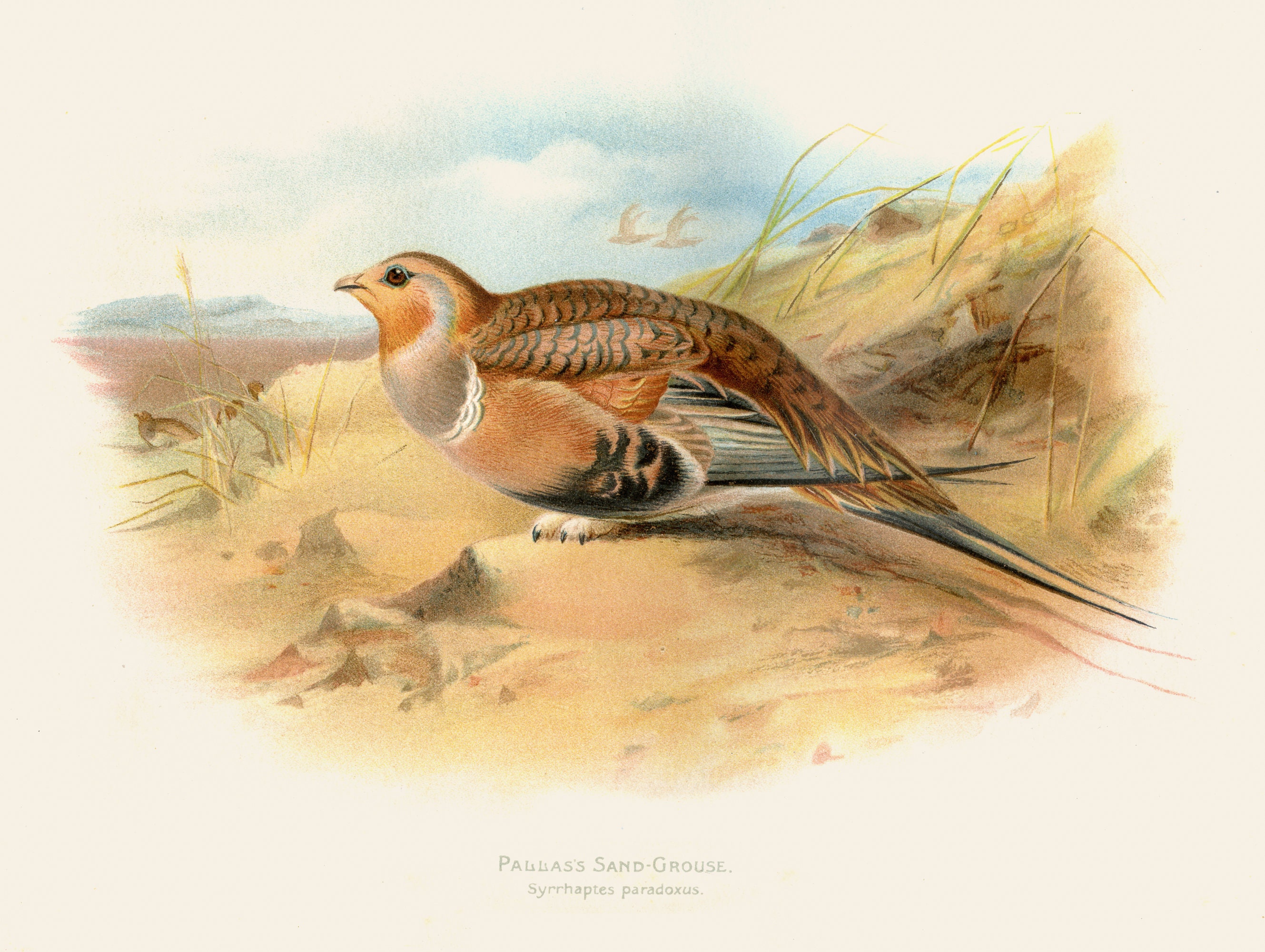The image is a detailed drawing of a Pallas’s sandgrouse (Syrrhaptes paradoxus). The bird is positioned facing the left, with its tail extending to the right. It is predominantly brown with distinct features: a crescent-shaped gray marking that extends to its eyes and some black markings, particularly on its wings and tail. The bird has a short beak and brown eyes. The underparts of the bird are tan with black markings, and the chest area shows a mix of gray and white.

The bird is perched on a sandy dune, with tufts of grass emerging sporadically from the sand. The background features a vivid blue sky adorned with gray and white clouds, suggesting a bright midday setting. Additional smaller birds are depicted in the sky, adding to the natural ambiance of the scene.

The entire scene, including the bird and the background, is encapsulated within an oval frame with faint edges, while the corners of the image remain white. Text at the bottom of the image identifies the bird with its common name, "Pallas's sandgrouse," and its scientific name, "Syrrhaptes paradoxus."